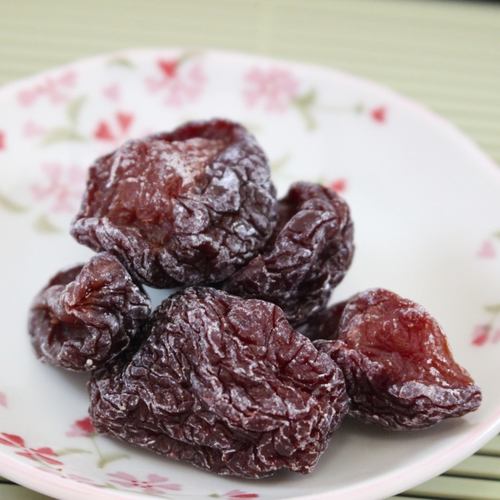The image features an arrangement of dried fruit, predominantly prunes, displayed on a white round plate adorned with pink and red floral patterns, including green leaves and stems. The prunes, numbering five in total, exhibit a variety of rich, dark hues ranging from deep purple to dark brown, with some lighter shades interspersed. The fruit pieces display a notably wrinkled texture, and two of the larger prunes have a slightly white coating, adding to their rustic appearance. The light green background provides a subtle contrast, drawing attention to the detailed floral design framing the fruit, with some elements slightly blurred to emphasize depth. The prunes are stacked on each other, creating a casual yet deliberate presentation.